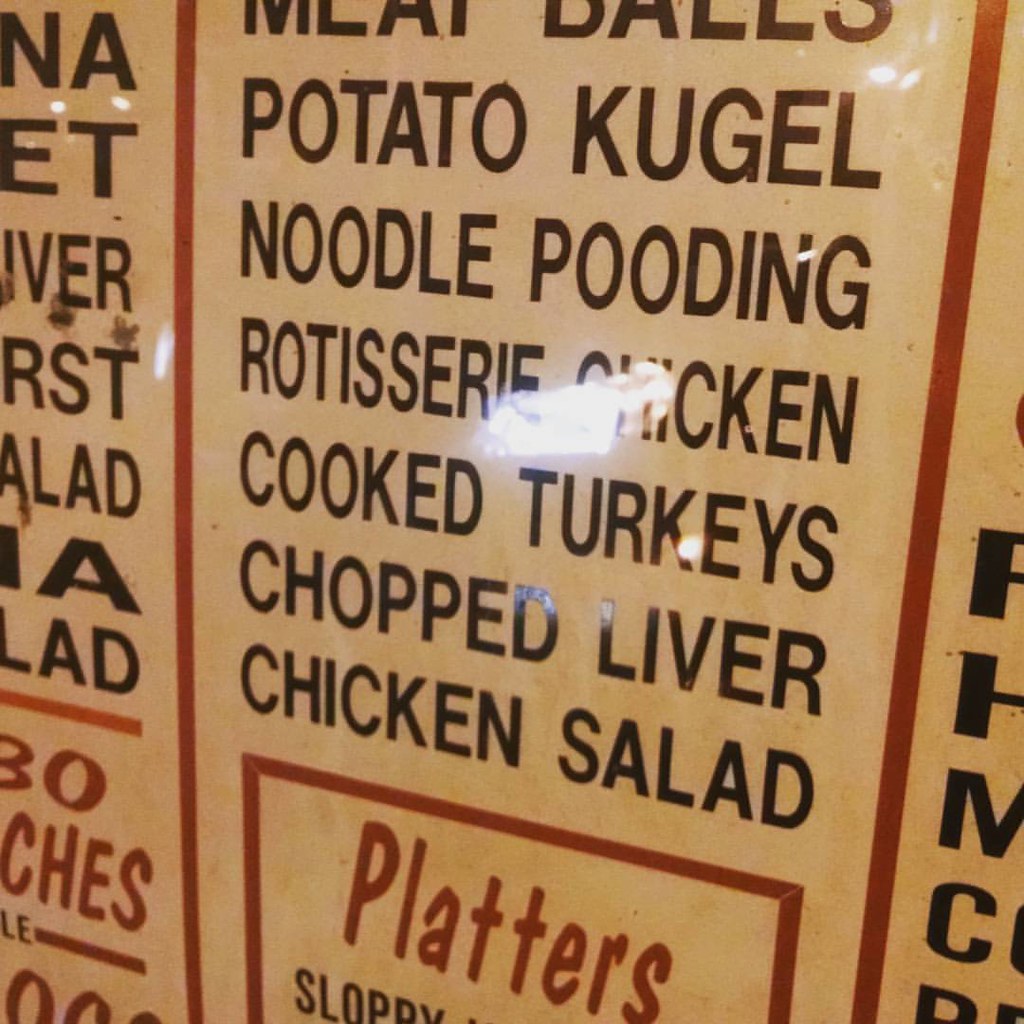The photograph depicts a large menu board, likely situated at the back of a fast food establishment, takeaway place, drive-in, or roadhouse. The menu is prominently displayed, making it easy for customers to read from a distance. The offerings listed include meatballs, potato kugel—a traditional Jewish dish made of savory potatoes—noodle pudding (though "pudding" is misspelled as "pooding"), rotisserie chicken, cooked turkeys, chopped liver, and chicken salad. Notably, the misspellings and the inclusion of Jewish cuisine suggest that the menu may originate from a country where English is not the primary language or possibly from an Israeli locale. The board appears to be a permanent fixture, either printed or painted, but clearly, some items were not spell-checked before its completion.